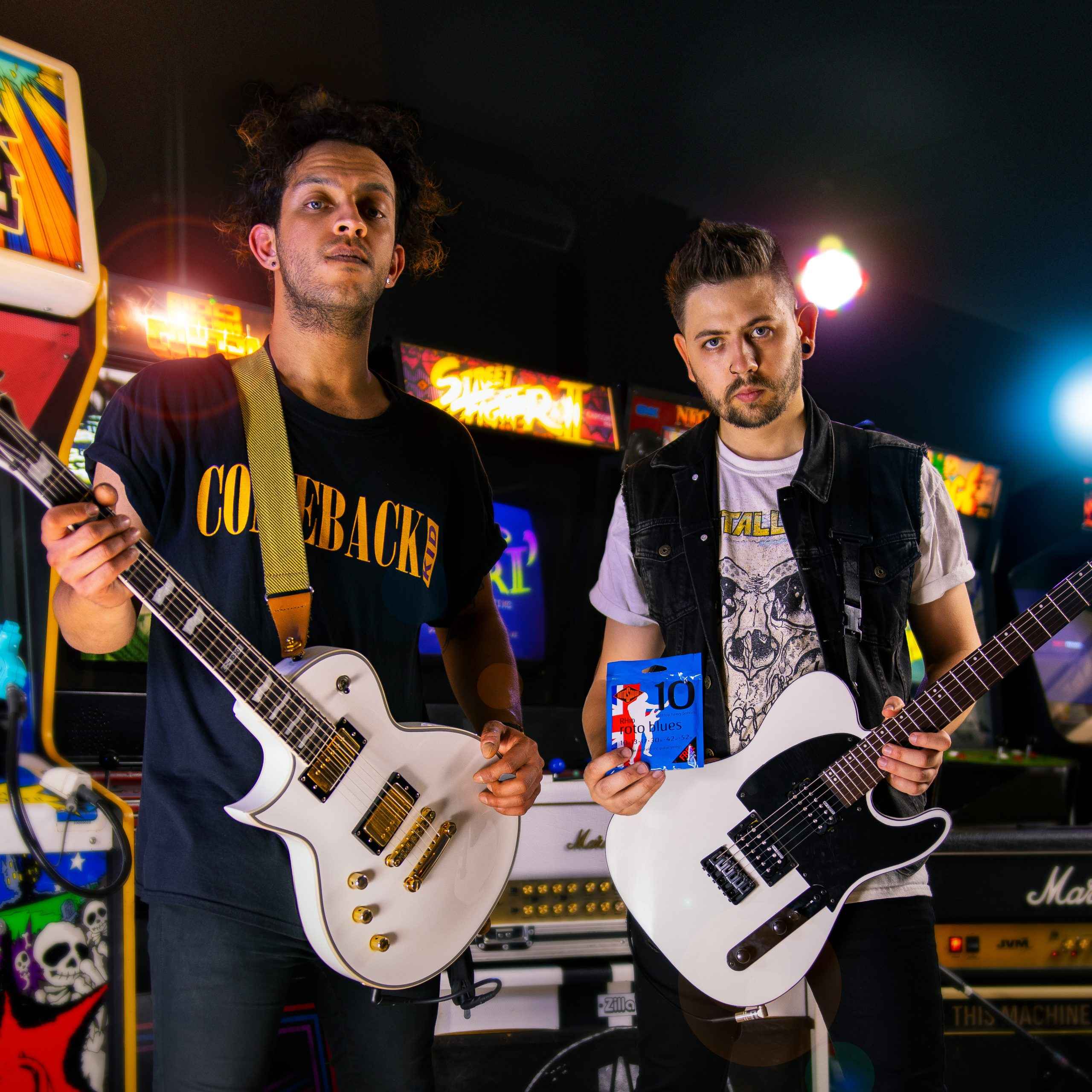The image features two men standing together, each holding an electric guitar. The man on the left is dressed in a black top with folded sleeves and black trousers. His shirt has the text "Comeback Kid" written in golden letters. He has medium-length hair stopping just above his ears, sports earrings, and exhibits stubble on his neck. He holds a predominantly white guitar with a black neck and golden highlights. The man on the right has styled, spiky hair and also wears earrings along with a beard. He is clad in a white shirt with a design in the middle—possibly a skeleton—and a sleeveless black jacket, paired with black trousers. His guitar is white with a black section on the body. Additionally, he is holding a small blue packet that says "Toto Blues" and has the number "10" on it. They appear to be in a well-lit arcade, with rows of arcade games like Street Fighter II and various equipment visible in the background, suggesting a lively atmosphere. Both men are looking directly at the camera.